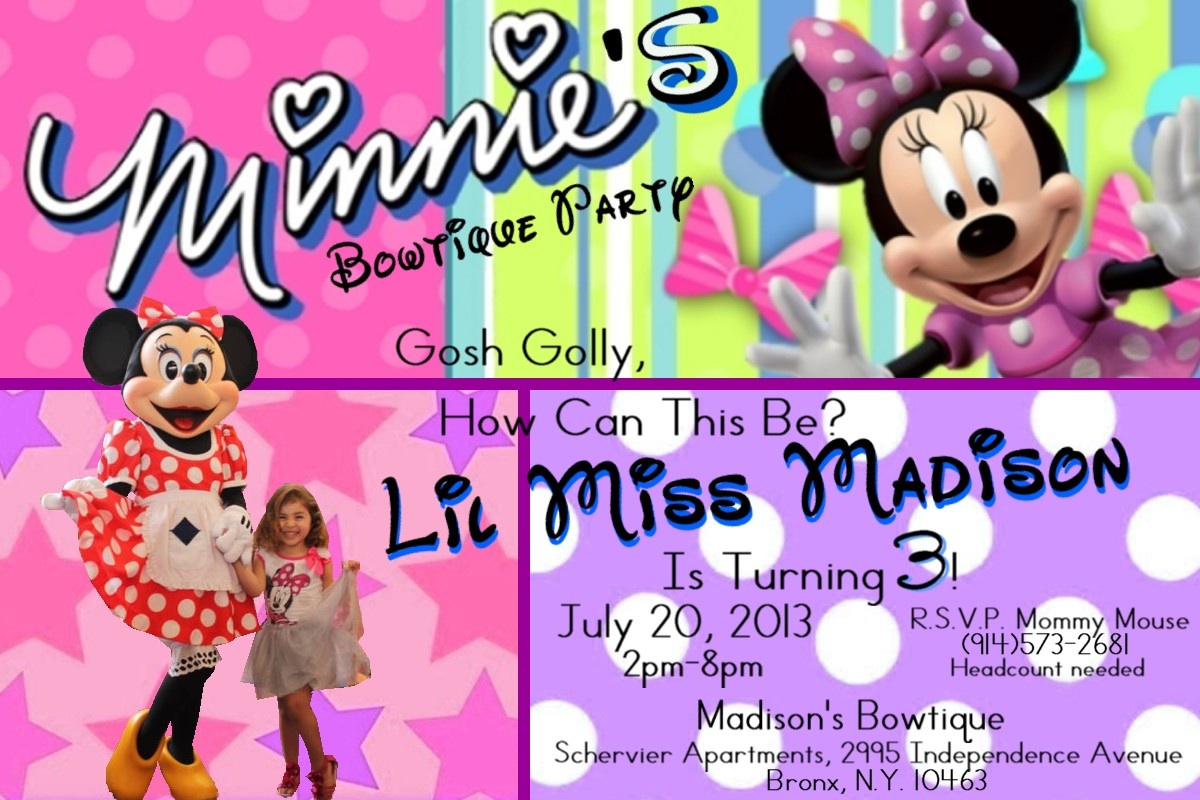This vibrant and colorful rectangular image serves as an advertisement for a Disney-themed birthday party. Across the upper left corner, the background is dark pink with lighter pink circular bubbles or spots, featuring the text "Minnie's Boutique Party" in a white, QT-style font outlined in black, angled upwards with heart-shaped eyes on the text. Adjacent to it, there is a longer rectangular section with vertical stripes in green, blue, and white. In the upper right corner, a 3D cartoon image of Minnie Mouse, adorned in her iconic pink and white polka dot bow with matching dress and black ears, grabs attention.

In the lower left corner, a young girl with long blonde hair, smiling and dressed in a Minnie Mouse outfit, stands against a pink background with dark pink and purple stars. She holds hands with another Minnie Mouse character clad in gold shoes, black leggings, a red and white polka dot dress, and a matching bow. In the center of the image, text reading "Gosh, golly, how can this be? Lil Miss Madison is turning three" is presented at an upward angle in black, highlighted in blue. Below, the details of the event are listed: "July 20th, 2013, 2 p.m. to 8 p.m. Madison's Boutique, Chervier Apartments, 2995 Independence Avenue, Bronx, New York, 10463. RSVP, Mommy Mouse, 914-573-2681. Head count needed." This section is set against a purple background with white polka dots, completing the festive invitation.